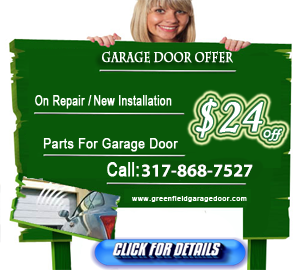This image is a screenshot of a simplistic, amateur-looking advertisement laid out in a landscape orientation. The centerpiece of the ad is a photoshopped image of a smiling young woman, likely in her twenties, with blonde hair and bangs. She has very white teeth and pink nail polish on her hands, which are positioned on either side of a green board graphic.

The text on this green board reads "THE TOP GARAGE DOOR OFFER" in bold, white, capital letters and is underlined for emphasis. Below this, the ad states, "On repair / new installation parts for garage door" followed by a phone number, 317-344-9291. There's a prominent notice of "$24 off" displayed in white text, enclosed by dual borders that make it stand out.

Toward the bottom of the advertisement, the website "www.greenfieldgaragedoor.com" is listed, and there is a blue button with white text that reads "Click for details."